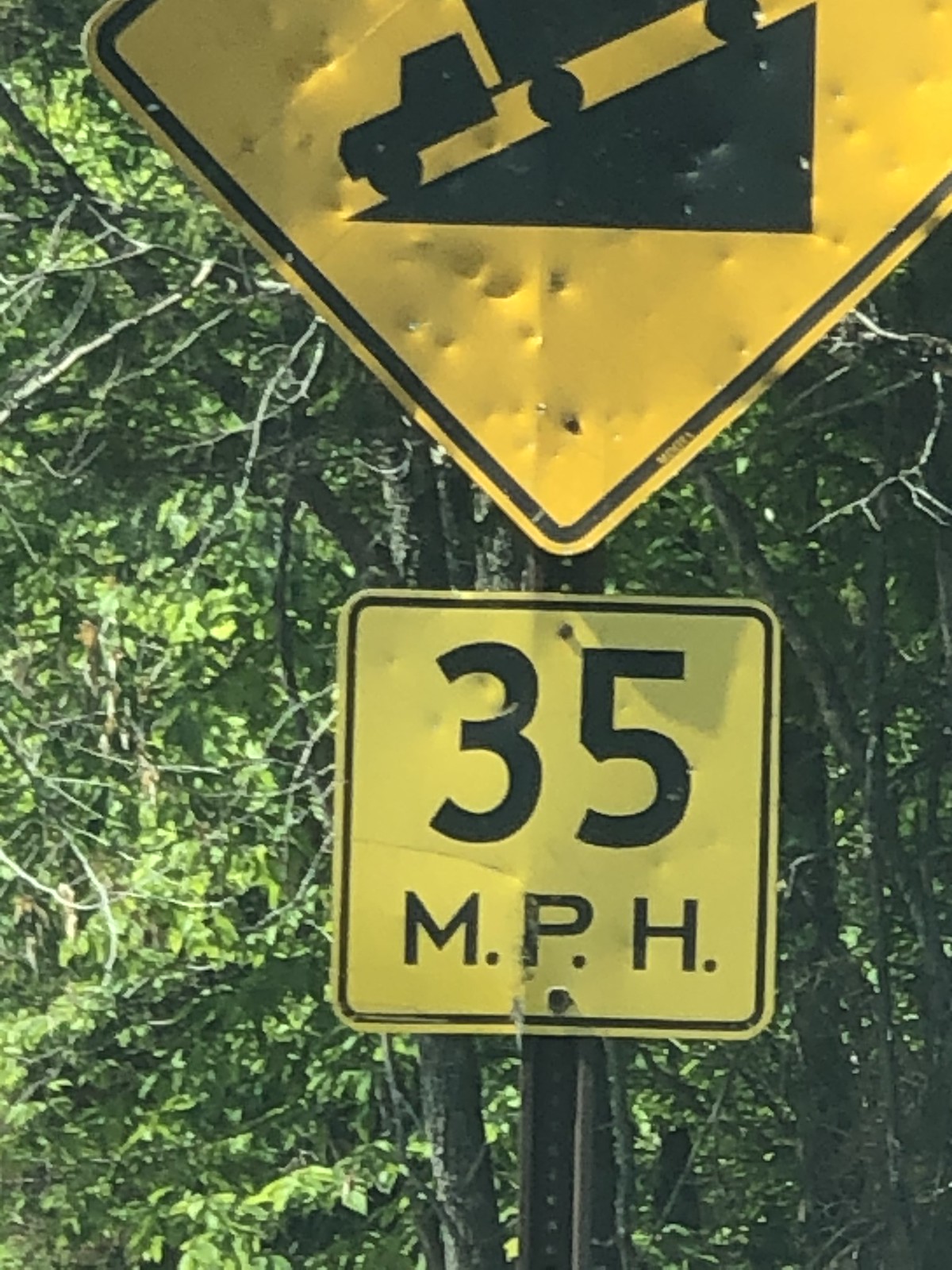The image shows a pair of damaged road signs mounted on a metal rod against a backdrop of lush green trees. The top sign is a yellow diamond-shaped caution sign, punctured with numerous dents and resembling bullet holes, illustrating a truck descending a steep, black triangular slope to warn of an incline ahead. Below it is a yellow, square speed limit sign indicating "35 MPH" in black font, also marked with visible dents and attached to the rod with black nails. The scene appears to be captured on a sunny day, suggesting someone zoomed in to take the photo, with trees, some bearing leaves and others with bare branches, framing the background.